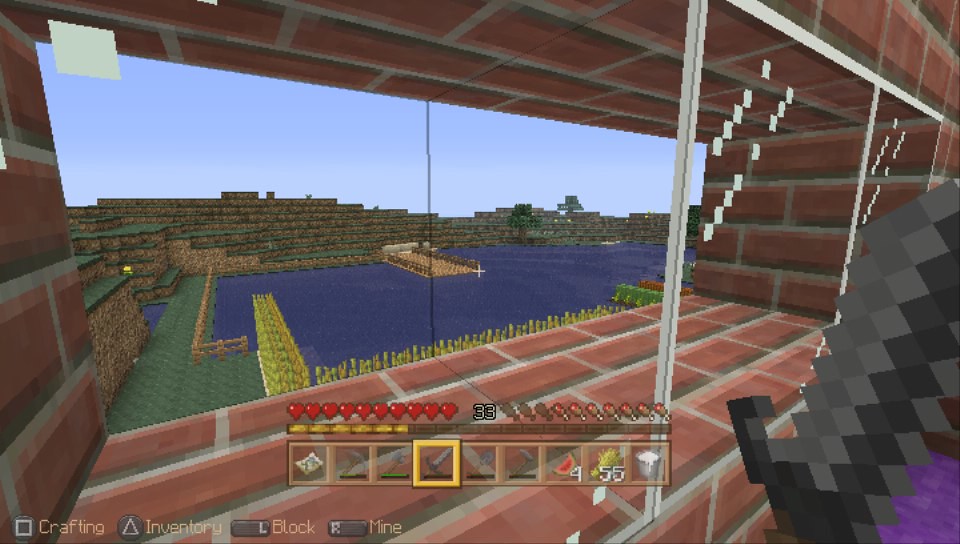In this rectangular image, we are looking at a screen displaying a scene from a video game. In the lower left corner, text reads 'Crafting', 'Inventory', 'Block', and 'Mine'. The scene features bricks arranged diagonally from the lower left to the upper right, extending upwards to form a wall, and then continuing across the ceiling, creating a brick enclosure. The front of this structure is open, allowing a view of other brick walls made from lighter brown stones rather than the red bricks.

Within this enclosure is a dark blue rectangular area of water, adding a rich, contrasting color to the scene. While no characters are visible in this segment, the lower right corner displays a zigzag pattern of black-gray blocks. This could possibly be the outline of a character's head seen up close, with a hint of dark purple in the lower right corner.

At the bottom center of the image, white text displays the number '455', which likely represents a score or timer. Additionally, the number '33' is visible, positioned between a row of hearts and a line of oblong, brown images, indicating gameplay statistics or resources.